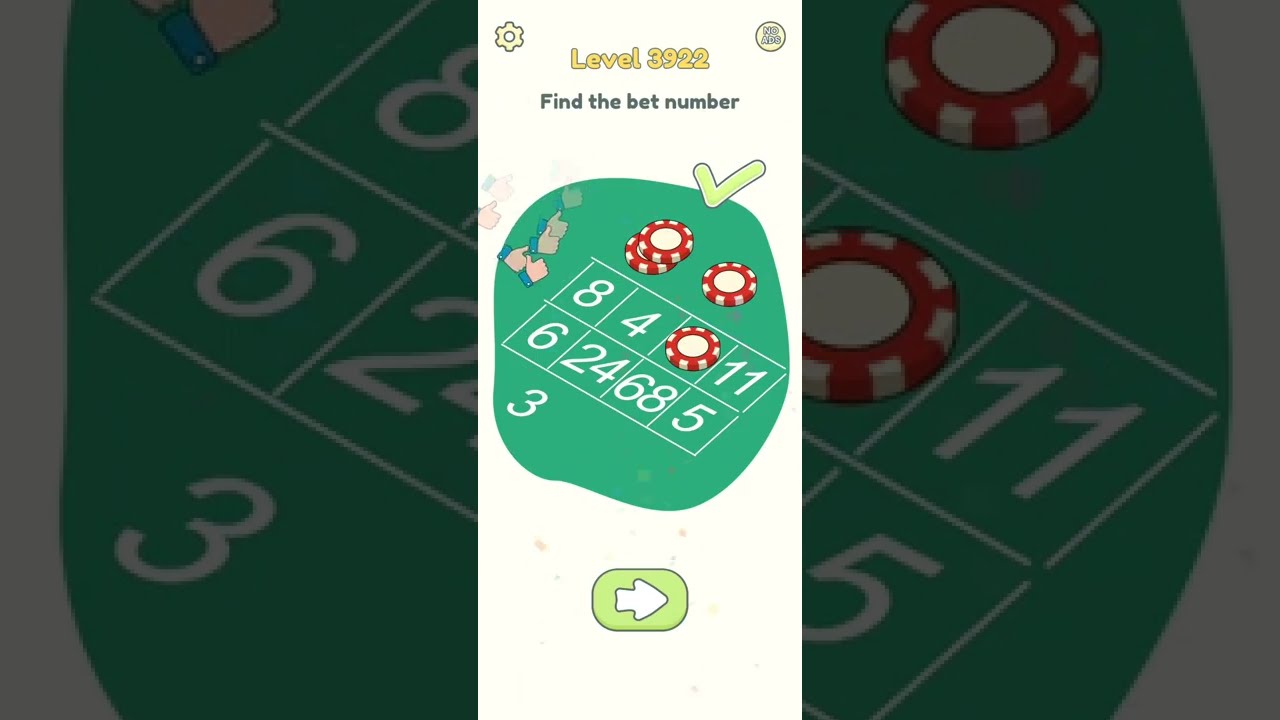This detailed image appears to be a digitally-created screenshot from a mobile gambling game, designed in a horizontal rectangular format split into three vertical sections. Dominating the center of the image is a betting table set against a black background, where various poker elements are meticulously arranged. The main text, displayed in yellow font, reads: "Level 3922, Find the bet number."

The central section is primarily white, containing a table marked with numbers including 4, 8, 11, 6, 24, 68, 5, and 3. Poker chips—red and white circles—are scattered across the table, resting on several of these numbers. Notably, the number 3 stands alone outside the white grid depicted on the table. Additionally, a lime green rectangle with a white arrow pointing to the right is positioned below the table.

The left and right sections of the image zoom in on parts of the table, showcasing more detailed views of the betting area. Specific numbers like 8, 6, 3, 11, and 5 are outlined in white squares, paired with poker chips. 

The overall scene is vividly colored with black, green, light green, yellow, white, and red hues, reinforcing the gambling theme. The layout suggests a task where the player must find a specific bet number, further emphasized by the central text directive: "Find the bet number." The presence of a settings icon and the level number signifies it as an app-based game.